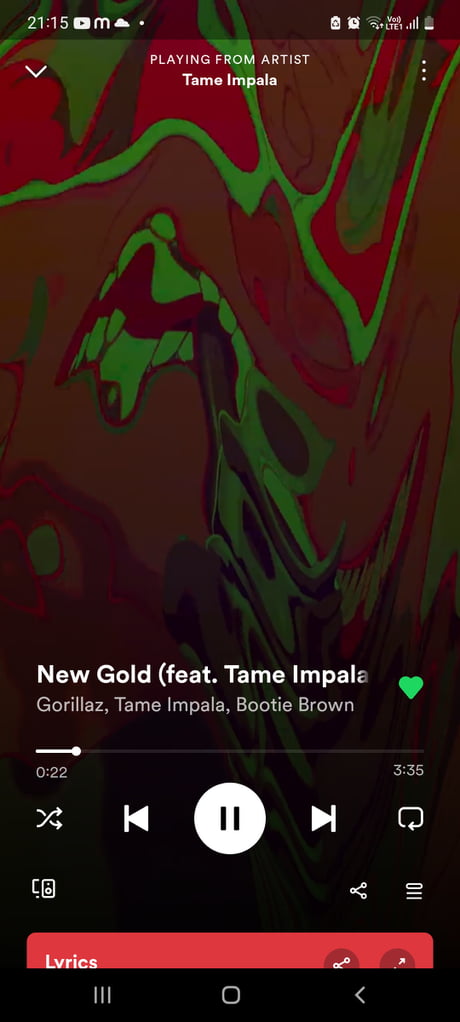The image displays a screenshot from a cell phone, showcasing a vibrant and abstract background dominated by a mixture of pea green, burgundy, and darker green hues, creating a beautiful, swooshy painted effect. At the top of the screen, the text reads "Playing from artist Tame Impala," indicating the music source. The song currently playing is titled "New Gold" and is attributed to multiple artists, listed as follows: "New Gold (feat. Tame Impala, Gorillaz, and Bootie Brown)."

In the "New Gold" section, a green heart icon is visible, suggesting it might be marked as a favorite. The song is 22 seconds into its total duration of 3 minutes and 35 seconds. Playback controls, including a pause button, forward and back buttons, and a continuous play button, are clearly displayed. Additionally, a prominent red button at the bottom of the screen features the word "Lyrics" in white print, indicating where users can click to view the song's lyrics.